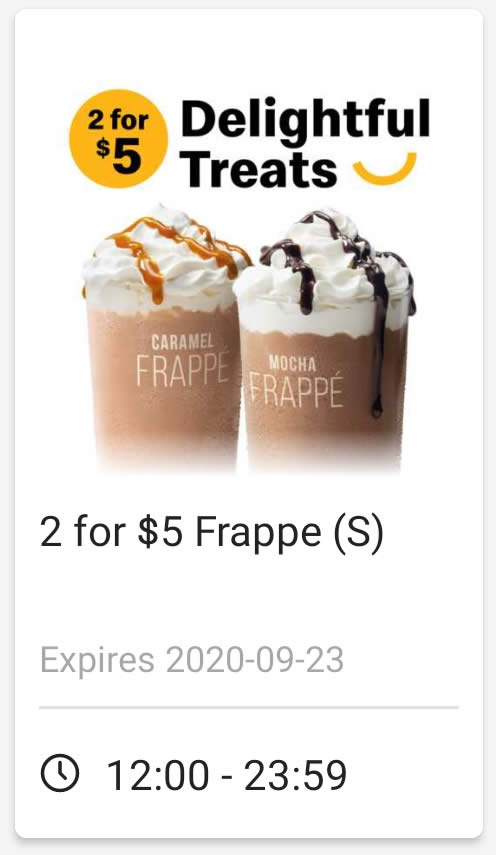On the left side of the image, there is a yellow circle with black text inside that reads "$2 for $5," accompanied by a small black dollar sign and the number five ($5). To the right of the circle, the phrase "Delightful Treats" is written in black text, next to a half-yellow circle. Below this text, an image showcases two coffee drinks. 

The first drink is a Caramel Frappé, characterized by its light brown base. It's topped with whipped cream generously drizzled with caramel sauce. To the right of this drink, the label "Mocha Frappé" indicates the second beverage, which has a slightly darker brown color. This Frappé is also topped with whipped cream, adorned with dark chocolate sauce in thin, dark lines.

Below the images of the drinks, the text reads "2 for $5 Frappé(s)" and underneath, in gray, it states "Expires 2020-09-23." A long gray line follows this text. Finally, there is an image of a clock, depicted as a circle with two small lines inside, next to the text "12:00 - 23:59."